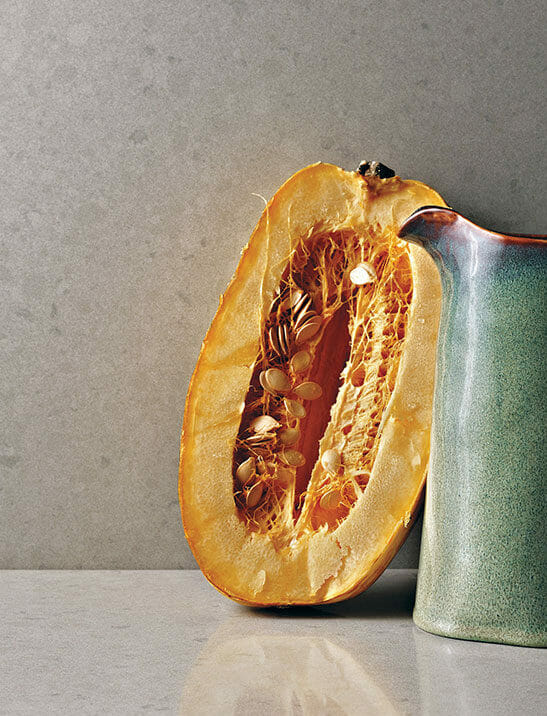This detailed color photograph captures a cross-section of a yellow-orange, oval-shaped squash or small pumpkin, prominently displayed against a gray background. The squash has been halved, revealing its fleshy interior filled with seeds and fibrous pith. One half of the squash leans diagonally against a tall, greenish-gray stoneware pitcher, adorned with a hint of red around the rim, located at the far right of the image. The scene is set on a shiny white, likely polished stone countertop, which reflects part of the squash at the bottom center of the photograph. The gray wall and glossy surface contrast with each other, accentuating the vibrant colors and textures of the vegetable and pitcher. The composition is free of any text, people, animals, or other man-made structures, focusing solely on the natural elements and their interplay with light and shadow.